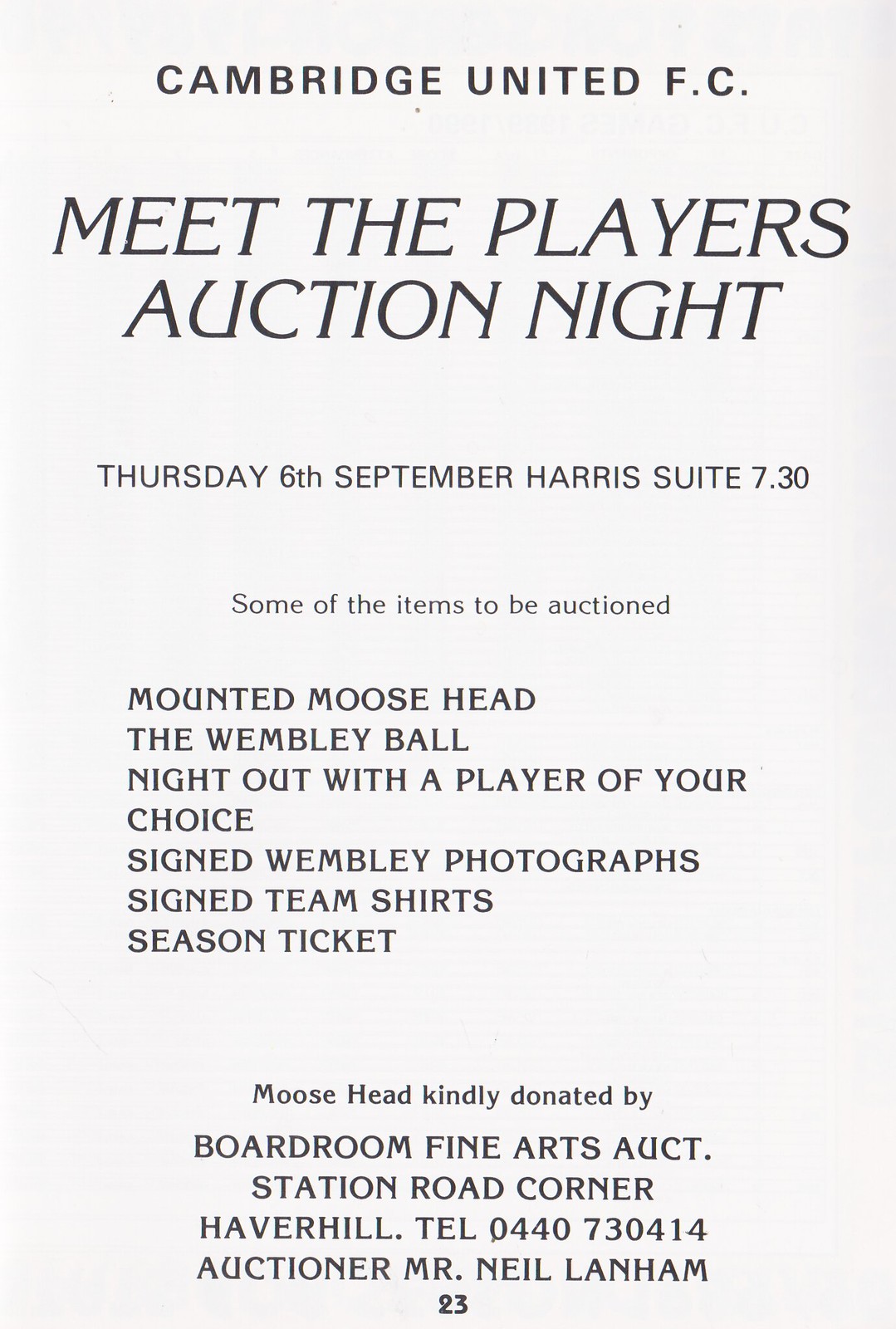The image is a detailed poster advertising an event. The background is light green with black text. At the top, it says "Cambridge United F.C." followed by "MEET THE PLAYERS AUCTION NIGHT" in capital, slanted text. Below, in capital letters, it states, "Thursday 6th September, Harris Suite 7:30." The poster then lists "Some of the items to be auctioned" including a mounted moose head (kindly donated by Boardroom Fine Arts), the Wembley ball, a night out with a player of your choice, signed Wembley photographs, signed team shirts, and a season ticket. The bottom of the poster provides the auction details: "Station Road Corner, Haverhill," the telephone number "0440 730 414," and mentions the auctioneer, "Mr. Neil Lanham." The number "23" is listed at the very bottom.